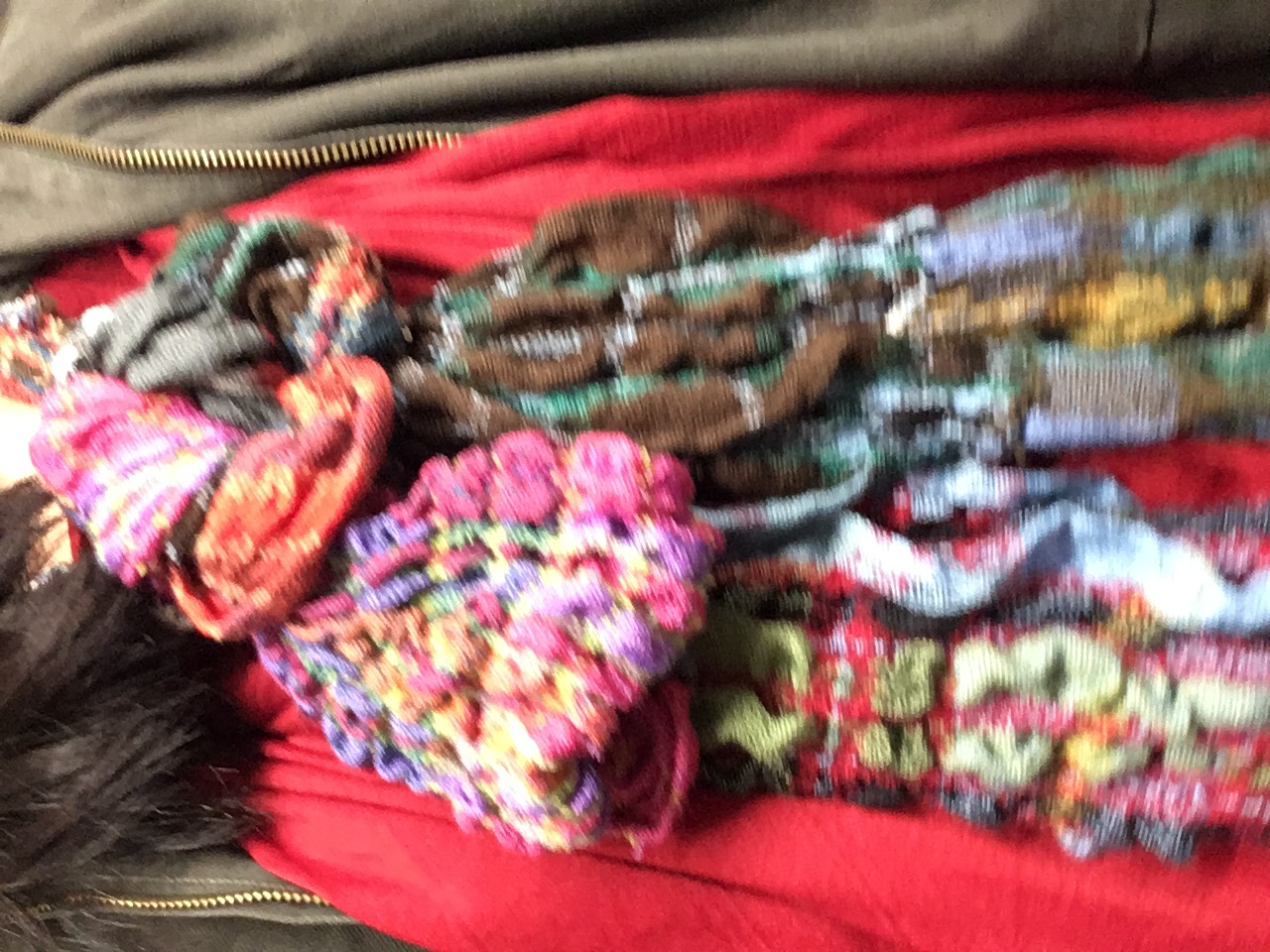In this slightly blurry photograph, the main subject is a striking, multicolored scarf draped over someone's chest. The scarf, embellished with a variety of textures and patterns, features an array of vibrant colors including brown, green, yellow, red, pink, and purple—almost resembling a tie-dye effect. Beneath this ornate scarf, a bright red, solid-colored scarf is visible. The person is wearing a brown zip-up jacket, with slight glimpses of their attire underneath—a green sweater layered over a red blouse. The image also captures the edge of their brown jacket and a strand of brown hair hanging into the frame from the top left, suggesting the presence of the person's head just outside the image's border. The overall composition creates a rich tapestry of colors and textiles, making the perspective appear somewhat confusing.